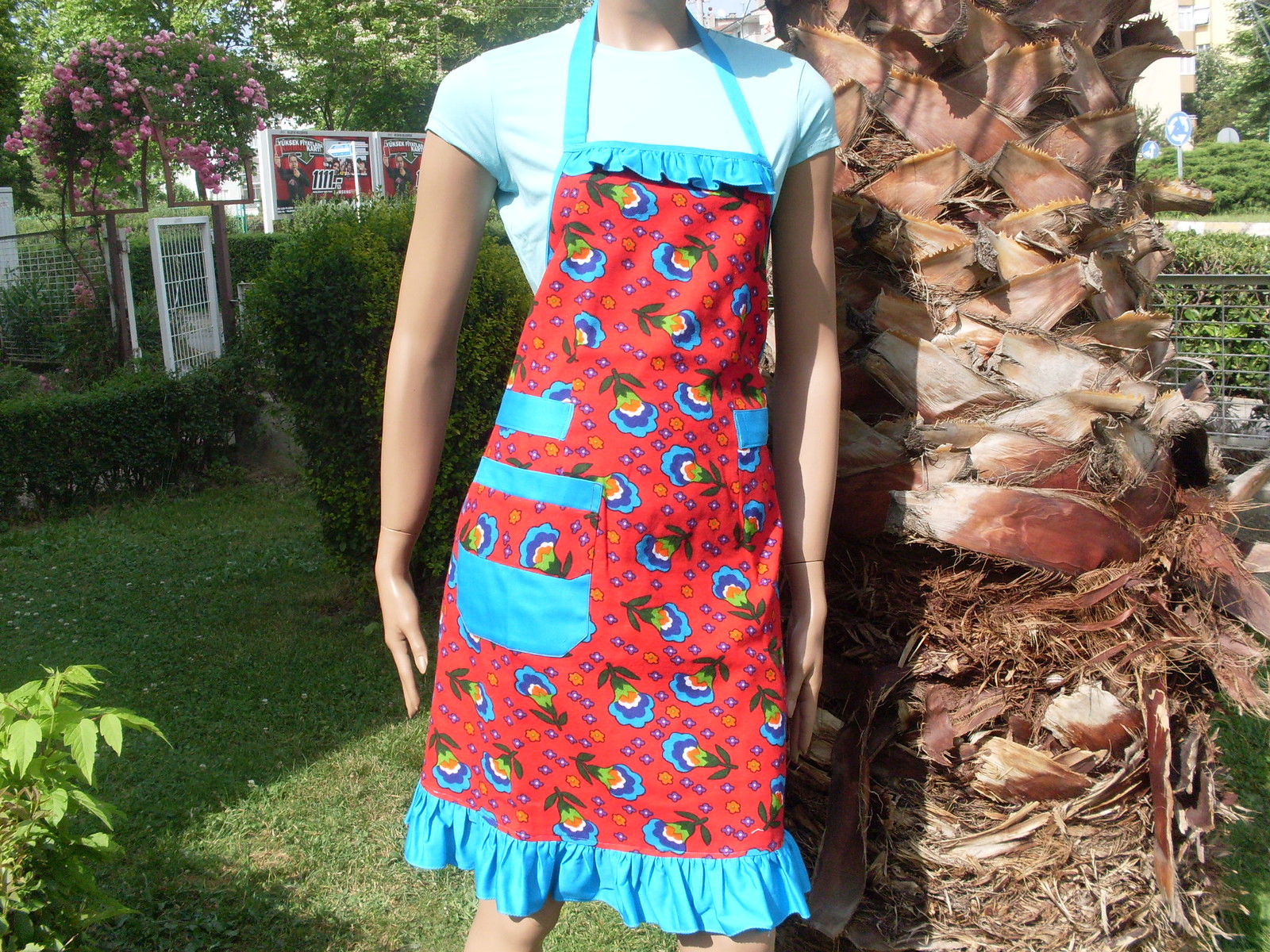The close-up image features a beige mannequin, identifiable by its stiff posture and plastic-like wrists and arms, standing in an outdoor setting. The mannequin is dressed in a short-sleeved light blue T-shirt, over which it wears a detailed apron. The apron has a light blue strap around the neck and a frilly light blue bottom edge. Its main section is predominantly red, adorned with a floral pattern that includes light blue, dark blue, yellow, orange, green, and white flowers, along with blue polka dots. The pockets on the apron have light blue edging. The backdrop includes a thick light brown palm tree trunk to the right, extensive green bushes, grass, and leaves behind and below the figure. On the left side, a tree with pink flowers is partially visible, along with a white gate topped by an arch covered in pink and green flowers, and a black metal fence in the distance. A hanging flower pot with light purple flowers is also seen in the background.